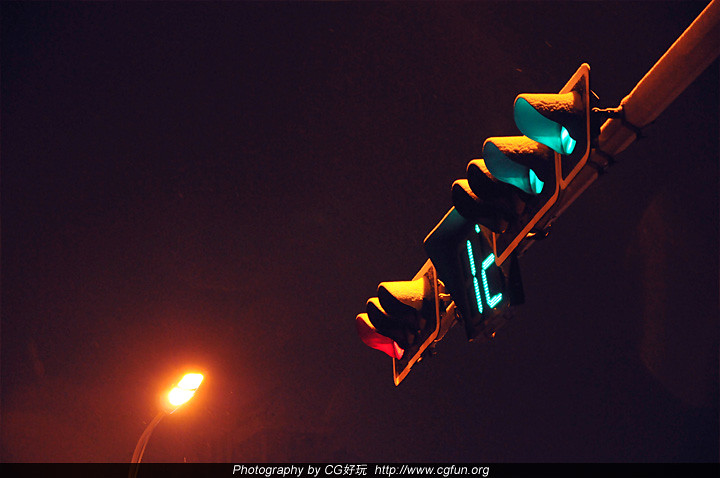This nighttime photograph, taken from a low angle, features a pitch-black sky devoid of any clouds or stars. Prominently displayed at the bottom of the image is the text "Photography by CG, http://www.cgfund.org." Dominating the left side of the image is a bright streetlight emitting an orange and yellow aura, mounted on a silver pole. On the right side, extending diagonally from the lower center to the upper right corner, is a traffic light. The traffic light displays the number "12" in a digital, greenish-blue font. Below this timer, a group of three lights shows a red light on the left, while above the timer, a second group of lights includes a pair of green lights on the right. The scene is an interplay of contrasting lights against an otherwise impenetrable night sky.